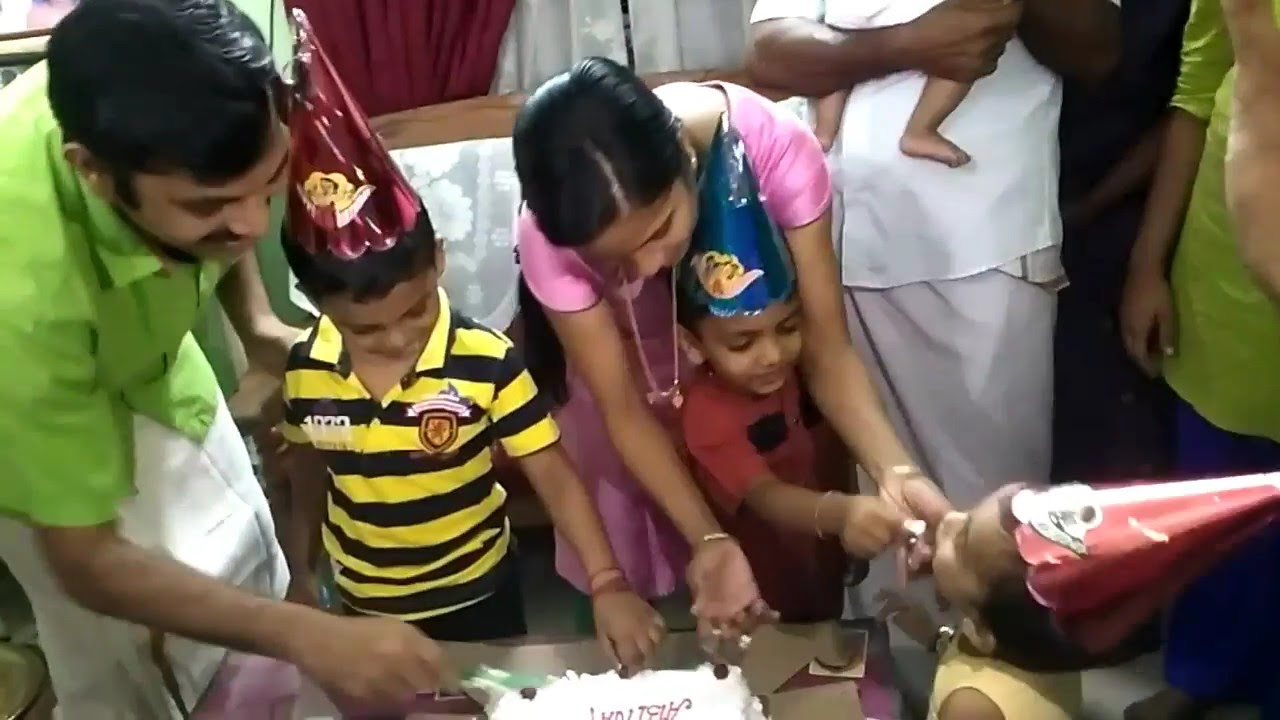In this image, capturing the warmth and bustle of an Indian family's birthday celebration, five main figures dominate the foreground. Central to the scene is a woman in a pink dress, with long black hair pulled back into a ponytail, leaning forward to feed cake to a small child wearing a blue conical birthday hat and a red shirt. This woman, possibly the mother, envelops the child with both arms, displaying a delicate necklace that dangles as she bends. Beside her, another young boy, likely her son, is engaged with the cake, wearing a black and yellow striped polo shirt and a red party hat. Adjacent to this child, a man believed to be the father, is bent over in a green button-down shirt and white pants, extending a hand towards the table with the cake. 

On the left side of the image, partly obscured, is a young girl in an orange shirt who is tilted up to be fed cake by her brother, wearing a red tank top and a party hat. In the lower part of the photo, a decorative birthday cake sits enticingly on the table. The background reveals the edges of more family members, with a woman dressed in white holding a baby, visible from the waist down, and another figure partially seen in a green shirt and blue pants. The scene is set in a cozy living room, as suggested by the glimpse of a red curtain in the distance, adding to the intimate, joyful atmosphere of the celebration.